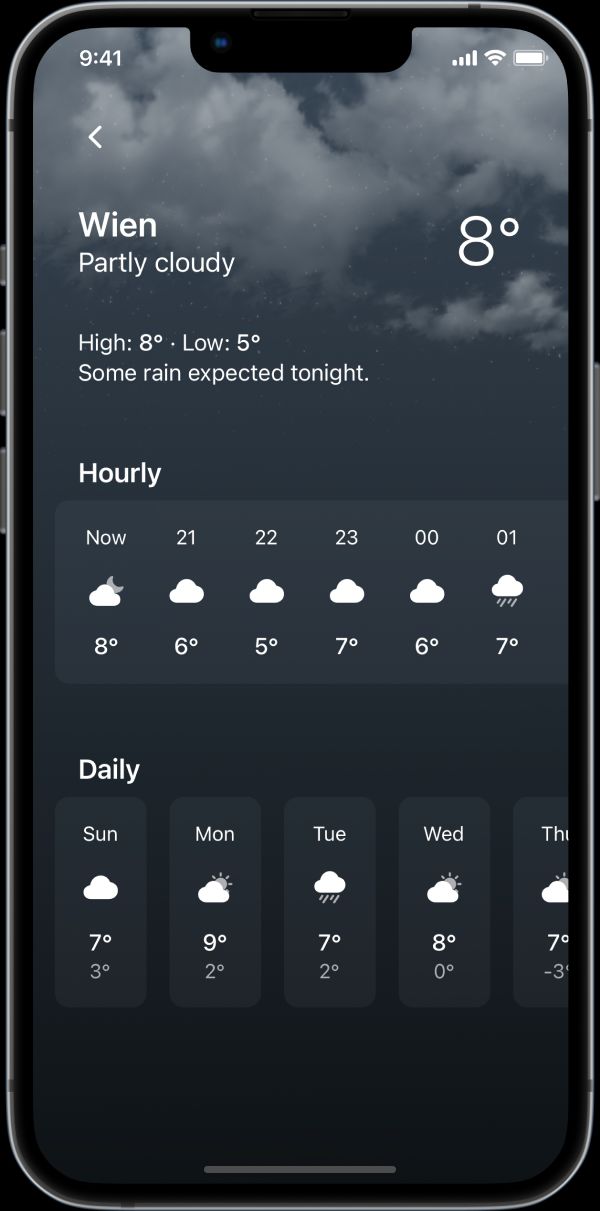The image showcases a weather app page on a smartphone. The background transitions from a dark blue sky adorned with light grey clouds at the top, to a solid dark blue at the bottom. Positioned prominently at the top left is a large white icon, likely representing weather conditions. Below the icon, the location is displayed as Wuhan with a current weather status of "Partly Cloudy."

To the right of this information, the temperature is indicated as 8 degrees Celsius. Just beneath the "Partly Cloudy" text on the left, high and low temperatures are listed: a high of 8 degrees and a low of 5 degrees. An additional note forecasts "Some rain expected tonight." The text throughout the app is written in white for clear visibility.

Lower down, an hourly weather forecast begins with "Now: 8 degrees, cloudy." Following this, at:

- 21:00 — 6 degrees, cloudy
- 22:00 — 5 degrees, cloudy
- 23:00 — 7 degrees, cloudy
- 00:00 — 6 degrees, cloudy
- 01:00 — 7 degrees, some rain

Beneath the hourly forecast is a "Daily" section providing an extended outlook:

- Sunday: 7 degrees high, 3 degrees low, cloudy
- Monday: 9 degrees high, 2 degrees low, partly cloudy
- Tuesday: 7 degrees high, 2 degrees low, rainy
- Wednesday: 8 degrees high, 0 degrees low, partly sunny
- Thursday: 7 degrees high, -3 degrees low, partly sunny

The clouds and partially sunny icons are displayed in white, matching the text color throughout the app.